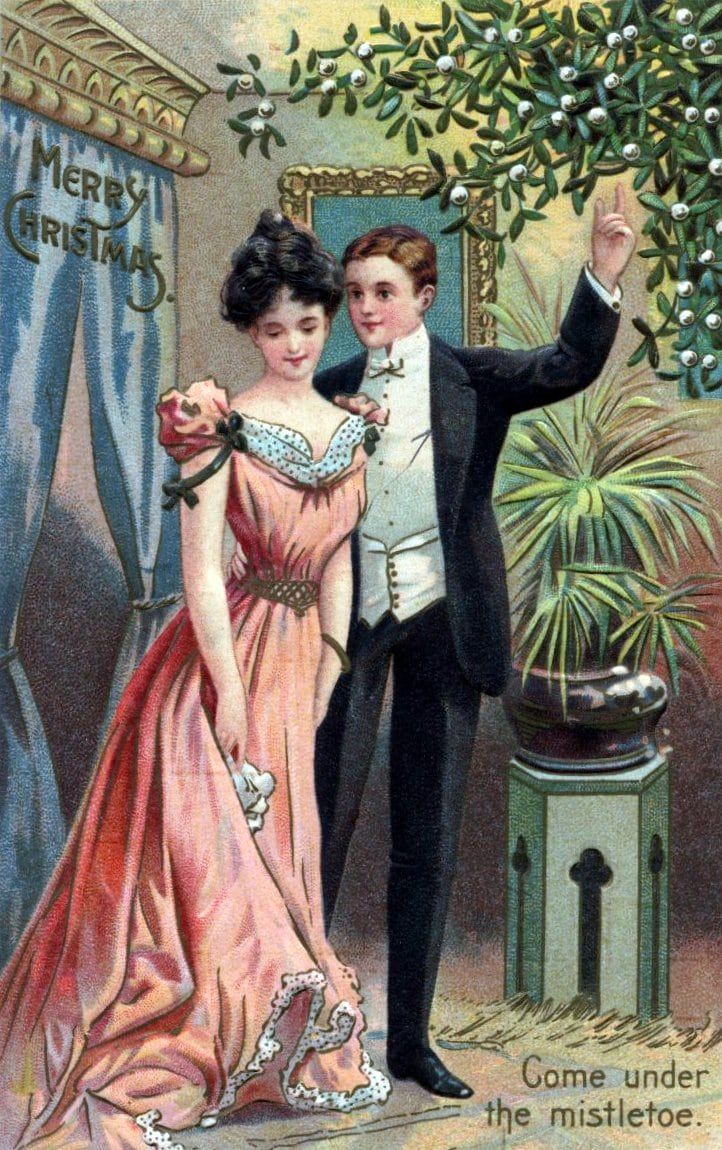The image resembles an old-fashioned Christmas card, possibly from the 1920s or 1930s. It features a man and a woman standing under mistletoe, with festive greetings and decorations enhancing the nostalgic feel. In the bottom right corner, the phrase "Come under the mistletoe" is written in an evergreen color, while "Merry Christmas" appears in the top left corner against blue curtains. 

The man, a white male with short reddish-brown hair, is dressed in a black tuxedo that highlights a white cummerbund and bow tie. He stands with his arm around the woman, who looks down shyly. She is dressed in a floor-length, peach-toned gown featuring a V-neck with a flower on the shoulder and a filigree belt at her waist. Her dark hair is styled up in a bun, with curly fringes falling over her forehead. She holds white flowers in her right hand. 

In the background, there is a potted plant on a pedestal, and a partial view of a tree adorned with silver ornaments can be seen in the top right corner. The quaint setting, including the gold cornice above the curtains, harks back to an era of old-time Christmas cheer.